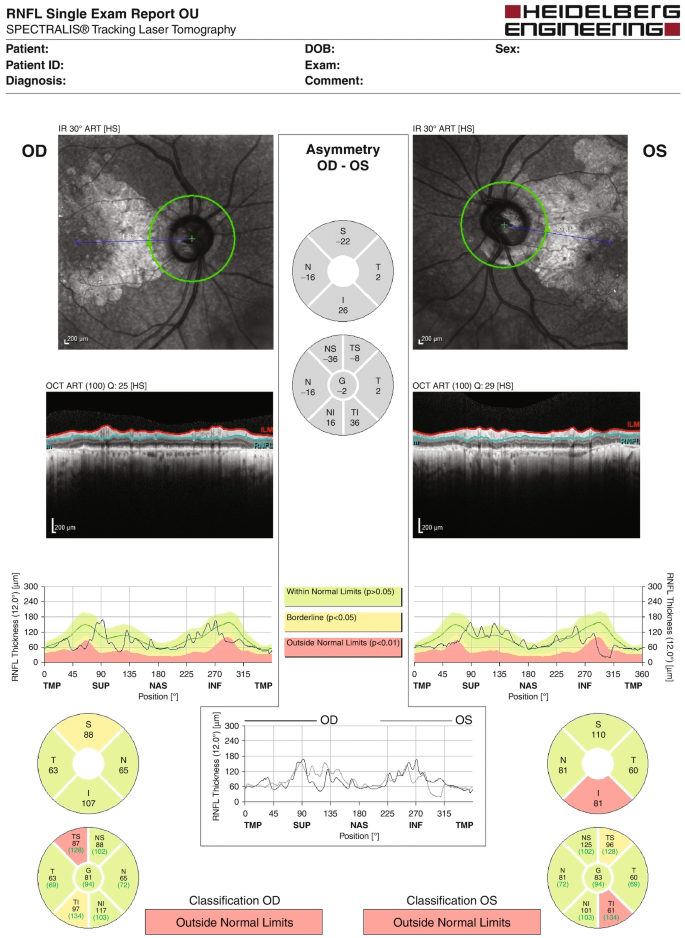This image is a detailed medical diagram associated with an eye exam, produced by Heidelberg Engineering. At the top, the text reads "Heidelberg Engineering," followed by the title "RNFL Single Exam Report OU, Spectraless Tracking Laser Tomography." Beneath this title, there is a section designated for patient information, which includes fields such as Patient, Patient ID, Diagnosis, Date of Birth, Exam, Comment, and Sex, though these fields are currently blank.

The central portion of the image showcases two x-ray-like images labeled "OD" (right eye) on the left and "OS" (left eye) on the right. Between these, the text "asymmetry OD-OS" indicates a comparison between the two eyes. Below these images, there are graphs that assess the functioning of different parts of the eye. The graphs are color-coded, with green signifying within normal limits, yellow indicating borderline, and pink representing outside normal limits. The numbers on these graphs range from 0 to 300.

Additionally, at the bottom, there are pie-chart-like circles that visually represent further diagnostic information. These charts use the same color coding to indicate normal limits, borderlines, and abnormalities. The overall presentation is a comprehensive visual report derived from laser tomography, emphasizing the detailed analysis of eye health without depicting any humans or animals.